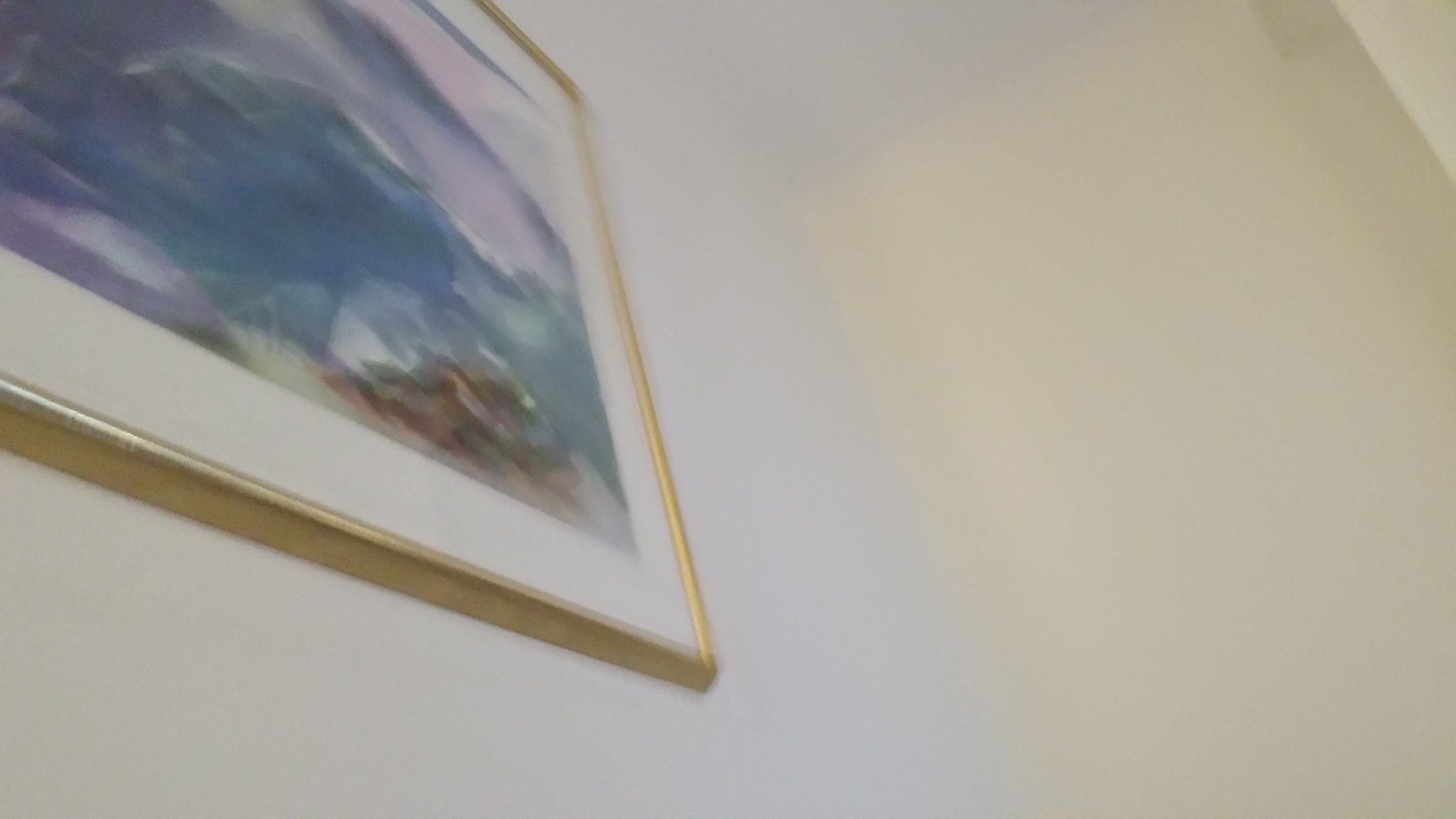The image depicts a blurry corner of a gold-framed painting mounted on a very light beige or light gray wall, with the camera angled upwards towards the frame. The frame is bordered by a white matting, inside which lies a blue-dominated artwork, possibly a watercolor, depicting an underwater scene. The picture features hues of blue and some purple, with bubble-like elements scattered about. There's a notable brown section in the lower right corner that seems to resemble a rock or a cluster of brown feathers, surrounded by dark blue and touches of black, giving the impression of ocean waves crashing against it. The right side of the painting fades into white caps and possible shoreline sand, creating a dynamic, wave-rich vista. The left side of the picture is not visible in the image. Additionally, part of the ceiling appears on the right-hand side, transitioning from the wall's color to a tan shade.